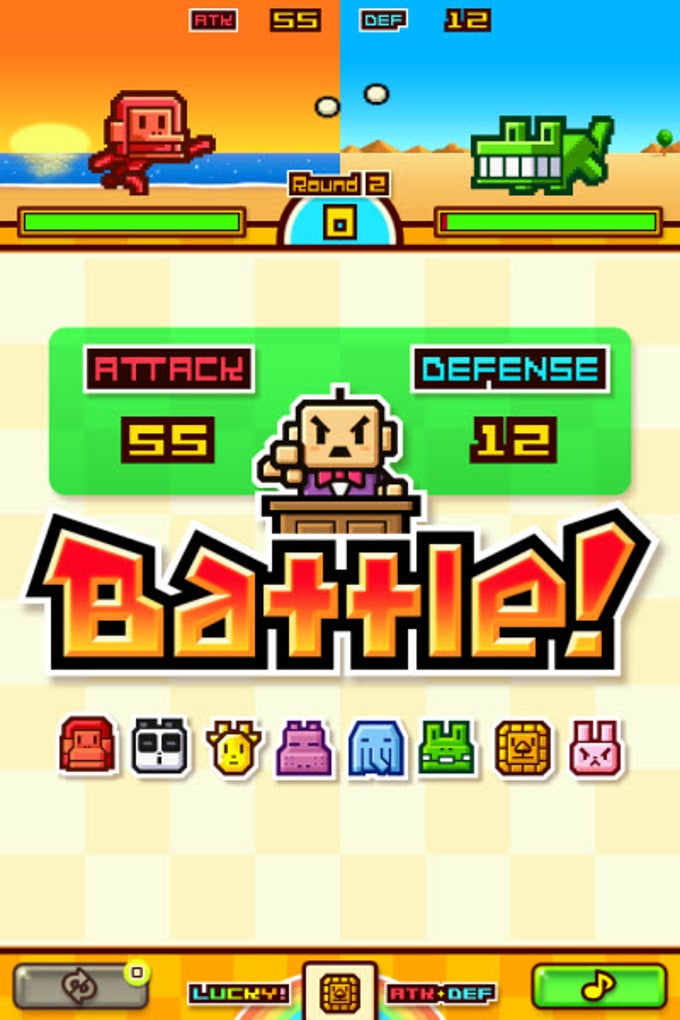In this mobile video game screenshot, the main focus is a vertical rectangle interface displaying a classic, arcade-style game. Dominating the center of the screen is a blocky robot character dressed in a purple suit and red bow tie, poignantly pointing towards the player with a seemingly angry expression. The word "Battle" is emblazoned across the screen in bold text, with the top half in red and the bottom half in a yellow-orange gradient. Below this, the game's score reads "Attack: 55, Defense: 12," suggesting a gameplay scenario.

In the bottom right, a green button featuring a yellow music note icon stands out, while the bottom left hosts a grayed-out recycling icon. Additionally, the top section of the screen showcases two blocky animal figures: a green, cubist alligator-like creature on the right, and a red monkey on the left. This imagery, combined with the primitive graphics and the array of colors including red, orange, yellow, green, blue, purple, pink, beige, black, white, and gray, evokes a nostalgic feel reminiscent of 70s or 80s video games.